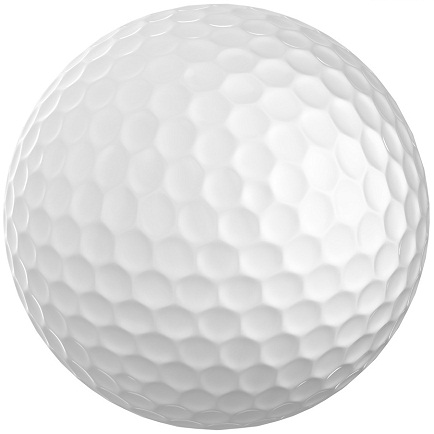This high-resolution photograph showcases a pristine, white golf ball against a white background. The golf ball features the typical concave dimples, predominantly hexagonal in shape, reminiscent of a Callaway design, though it bears no logo. A few smaller pentagon-shaped dimples are scattered to ensure complete coverage. Professional lighting techniques create an even illumination with highlights and reflections concentrated on the right side of the ball, while the bottom appears slightly shadowed, enhancing its three-dimensional appearance. There are no other notable features or distractions in the image, making the simplicity and detail of the golf ball the focal point.